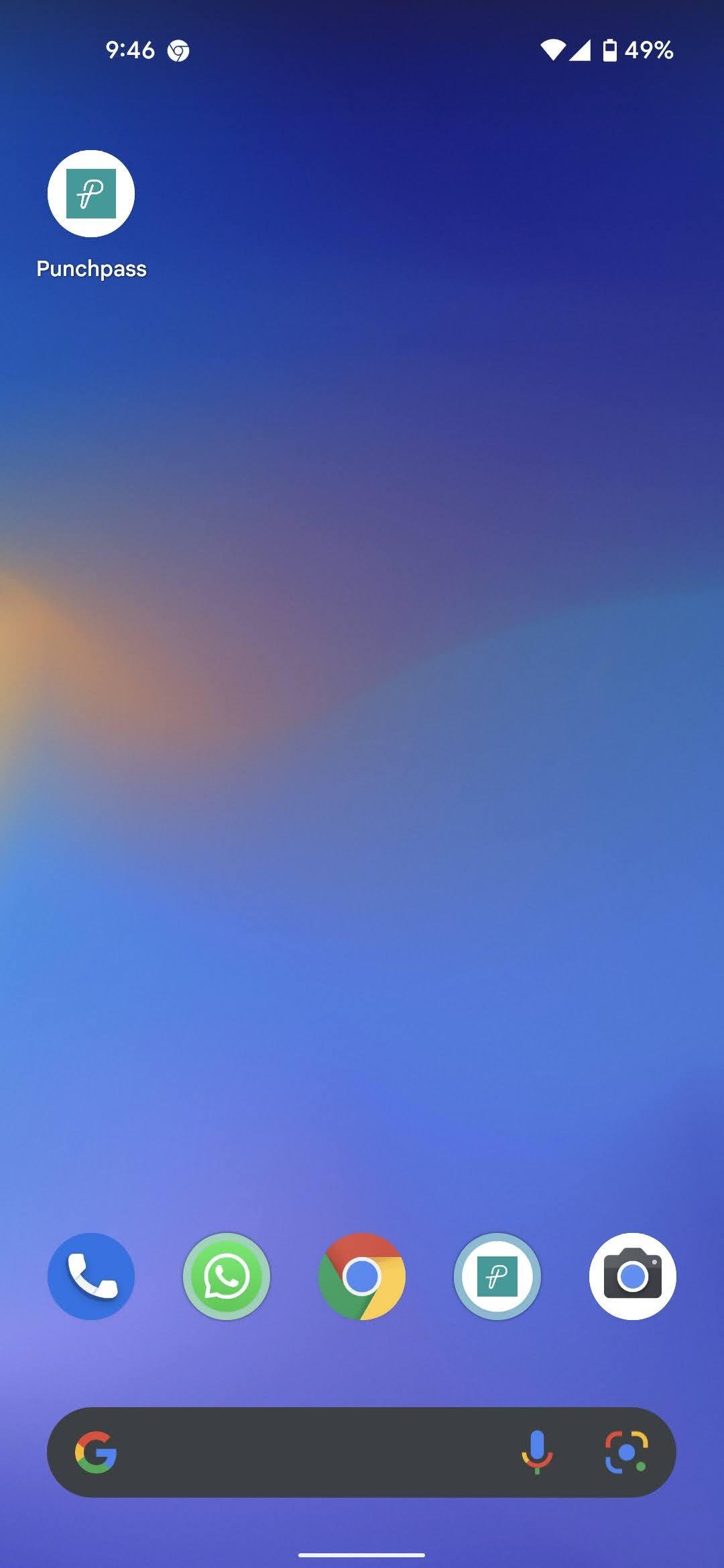A detailed and cleaned-up caption for the described cell phone screenshot would be:

"The screenshot displays a cell phone home screen with a gradient background transitioning from a black top through shades of dark blue, purple, orange, green, light blue, and finally light purple at the bottom. In the upper left corner, the time is shown in white text, accompanied by a small white icon to its right. The upper right corner houses icons indicating battery level, reception, and Wi-Fi strength. Approximately five lines down from the top on the left side, there's an icon labeled 'Punch Pass' in white, after which the screen remains blank until the bottom.

At the bottom, the navigation bar features several icons from left to right: a green phone icon, a blue text messages icon, a circular Chrome browser icon, followed by an unidentified white icon with a green square housing a white knot-like symbol, then a camera icon. Below these, spanning the bottom of the screen, is a black long oval containing a Google 'G' icon on the left and an icon for a microphone on the right."